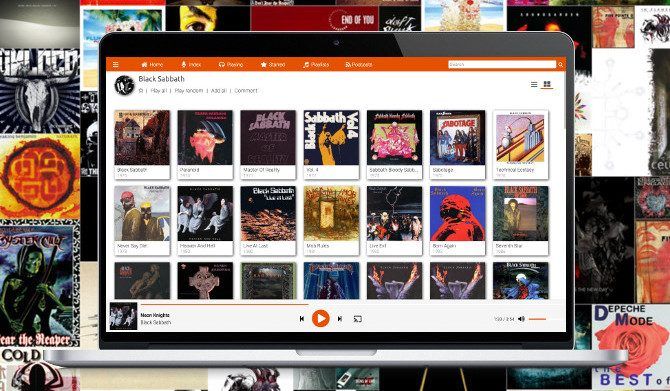The screenshot showcases a multi-layered visual with two distinct sections. 

In the background, extending across the whole frame, there is an image featuring several music albums. Prominently visible in the bottom right corner is "The Best of Depeche Mode" album. On the bottom left, there appears to be a Coldplay album cover. At the upper center of the background, there's another image, though it's not clearly identifiable.

Overlaid on this backdrop, a digital representation of a laptop occupies the forefront. The laptop itself has a silver bottom right corner, and its screen is framed in black. An orange stripe runs across the upper left and right edges of the screen, beneath which the text "Black Sabbath" is displayed, indicating a page dedicated to Black Sabbath albums. The interface presented on the laptop screen features seven columns and three rows of Black Sabbath album thumbnails. Only a partial view of the third row is visible, suggesting the presence of a screen slider. At the bottom center of the screen, an orange play button is situated, and in the upper right, there's a faint silver line indicating a scroll bar for navigating further down the page. The currently playing song is by Black Sabbath and might be "Neon Knights."